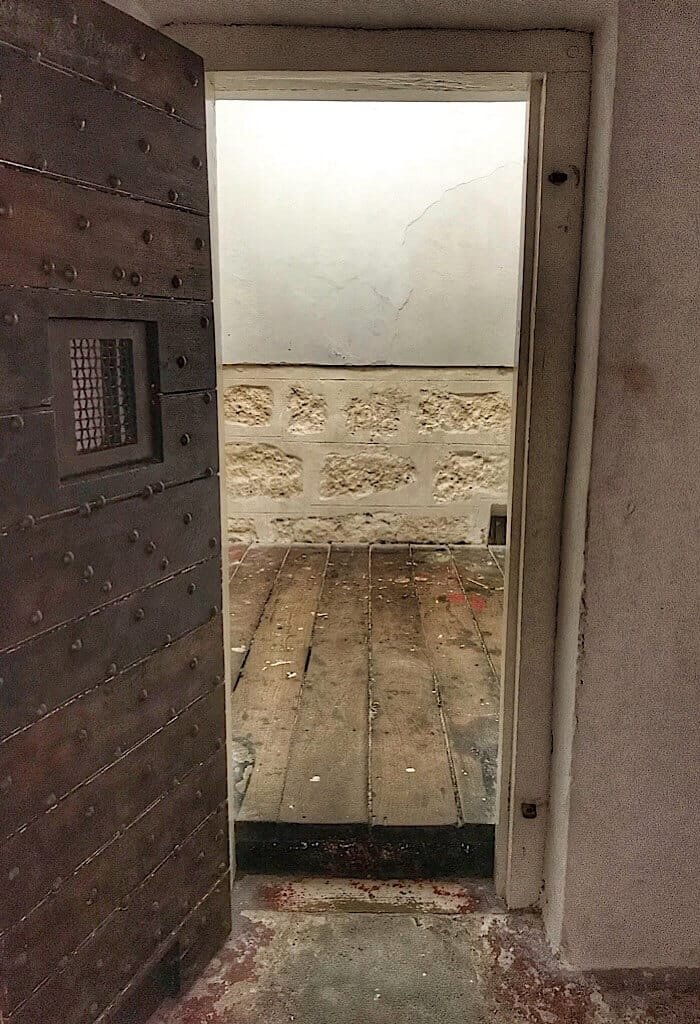The image depicts an interior of a room that closely resembles a prison cell or a dungeon in an old castle. The focal point is an old wooden door on the left, crafted from dark-stained wooden panels and reinforced with metal rivets. The door features a small metal grate or screen, likely used for monitoring the room's occupants. Adjacent to the door is a dark, worn brick wall leading to another wall facing the viewer. The room’s floor appears to be uneven, consisting of old, weathered wooden planks in varying shades from dark to light, indicating significant aging. The wooden floor transitions into a dirty, cracked, and partially painted concrete with red and gray hues. The walls inside the cell are possibly made of white-painted concrete or stone, showing signs of chipping and wear. There is a half wall or railing made of inlaid stone with visible grout. Beyond this railing, visibility is obstructed by a clouded, foggy view, enhancing the room's eerie atmosphere. Outside the open door lies a hallway lined with dark wooden panels, contrasting against a chipped, cream-white painted stone or concrete wall, topped with a layer resembling white plaster. The entire scene evokes the sense of an abandoned, possibly haunted fortress or detention area.